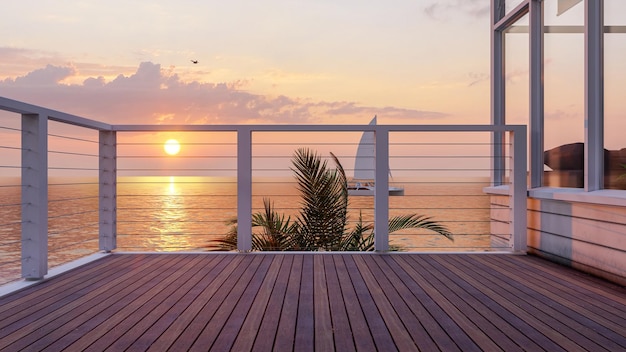The photograph captures a serene outdoor porch overlooking an expansive ocean, with the camera pointed directly at the water through the porch’s fence. The fence is constructed from cream-colored columns connected by horizontal parallel wires, and it wraps around from the front to the side, which is partially visible on the left. The building’s wall is partially visible on the right, and the room next to the porch is adorned with large windows. The wooden planks of the porch floor contrast with the metal wires of the railing.

Bathed in the warm hues of a setting sun, the scene radiates tranquility. The sun, positioned slightly above the horizon, casts a brilliant orange light across the water’s surface and into the sky, enhancing the atmosphere. The sun's vibrant glow creates an orange and yellow halo, with a gradient in the sky shifting from deep red to violet and lighter blue. Light cloud cover near the sun further enriches the sky with reddish-violet tones, while the rest of the sky remains mostly clear. In the bay, a solitary pontoon sailboat floats peacefully, adding a focal point to the ocean’s vastness. The very top of a palm tree peeks into view, contributing to the tropical ambiance of this picturesque seascape.